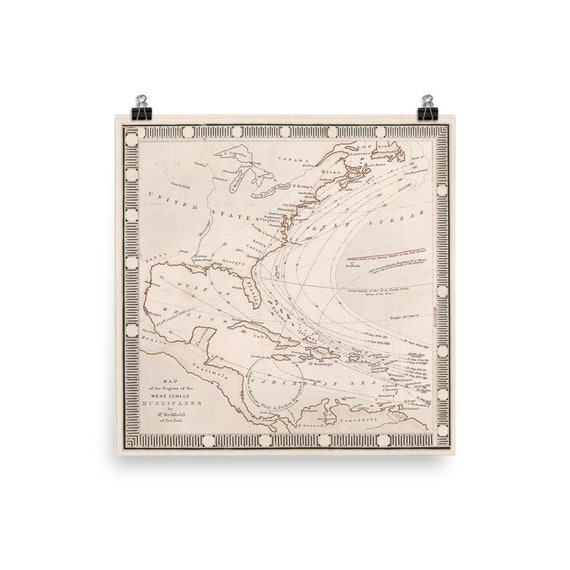A meticulously detailed map, secured to a wall with two clips, captures the viewer's attention with its intricate design and historical essence. Dominated by a circular motif, the map appears to depict a maritime region, possibly an ancient navigational chart. An array of tiny, precise script covers the map, demanding a closer look to discern the various annotations. Encircling the main map are several ornamental circular patterns, enhancing its antique allure. A prominent stamp, positioned centrally, suggests that this document has been authenticated, further hinting at its historical significance. The map highlights key geographical areas including the United States, Mexico, as well as the vast expanses of the Atlantic and Pacific Oceans. Rendered entirely in shades of pink, both the landmasses and their delicate contours create a visually striking, monochromatic study. The overall ambiance is one of vintage elegance and detailed cartographic craftsmanship.